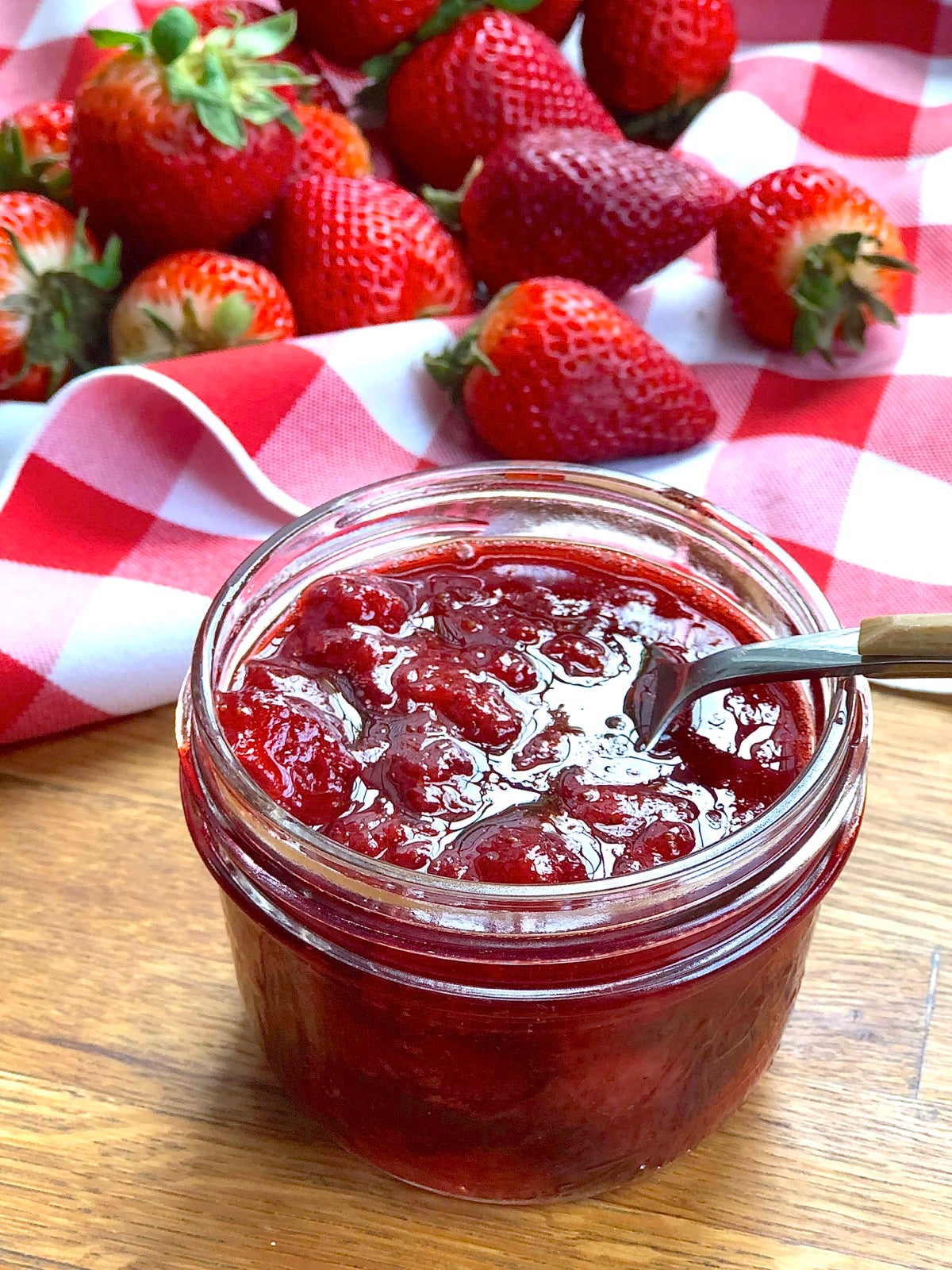The photograph is a carefully staged, close-up image taken indoors under artificial light, capturing a quaint, rustic scene. At the center bottom of the vertically rectangular frame, a small half-pint mason jar filled with liquidy strawberry preserves sits on a light wood surface, its grain and the lines between the boards clearly visible. A metal spoon with a wooden handle is inserted into the jar, extending towards the right but cut off at the edge of the image. Behind the jar, a red and white gingham tablecloth, reminiscent of an Italian restaurant, lays casually with visible wrinkles. Scattered atop this cloth are a heap of fresh strawberries, ranging in color from yellowish-orange, almost ripe, to dark red. The strawberries appear to have been nonchalantly strewn about, adding to the rustic charm of the scene.